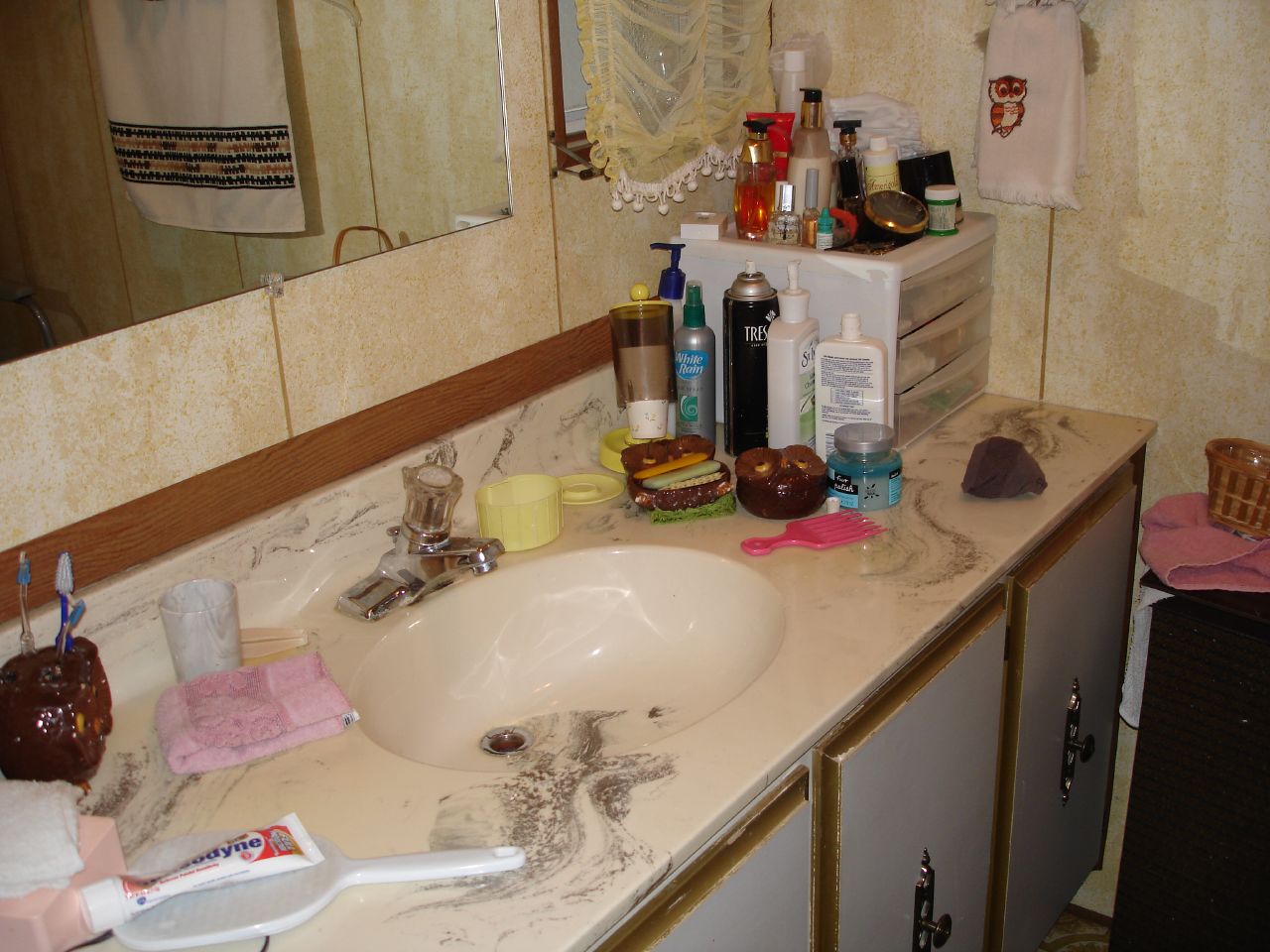The photograph captures the interior of a bathroom, specifically focusing on the sink and vanity countertop area, along with the cabinet underneath. The bathroom walls are adorned with decorative paneling in light tan and cream hues. A large flat mirror is affixed to the wall above the sink, reflecting the surroundings and adding depth to the room. Adjacent to the mirror is a small window that allows natural light to filter in.

The vanity countertop is spacious, stretching across a significant portion of the wall. It is made of a marbled material, adding an elegant touch to the space. The lower cabinets beneath the countertop are painted in a light color and are equipped with simple knobs for opening.

On the vanity surface, there are numerous personal care items neatly arranged. A white plastic-handled mirror lies face down, next to a tube of Sensodyne toothpaste. A red toothbrush holder, brimming with multiple toothbrushes, adds a pop of color. A neatly folded pink hand towel rests nearby. Additionally, there is a silver can of White Rain hairspray and a black can of TRESemmé hairspray, indicating a well-used and functional bathroom space.

This image encapsulates the essence of a well-maintained and everyday bathroom setting, complete with all the essential items for daily hygiene and grooming.